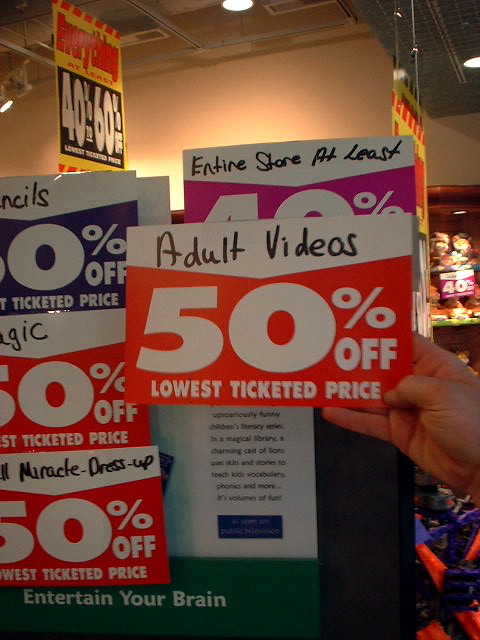The photograph is a vertically-oriented, slightly dimly-lit image taken inside a large store with tall ceilings. The focus of the image is on a succession of paper sales tags positioned towards the front, specifically on the left side, moving from the center to the bottom of the frame. Prominently in the center, a man is holding up a white sign with bold black text that reads, "Adult Videos, 50% Off, Lowest Ticketed Price." Surrounding this sign are additional labels in red, blue, and pink hues. To the right of the man, shelves stocked with various items can be seen. The lighting in the store comes from recessed fixtures in the ceiling, adding to the overall ambiance. In the lower left corner of the image, beneath the line of tags, a poster with the slogan "Entertain Your Brain" is visible.